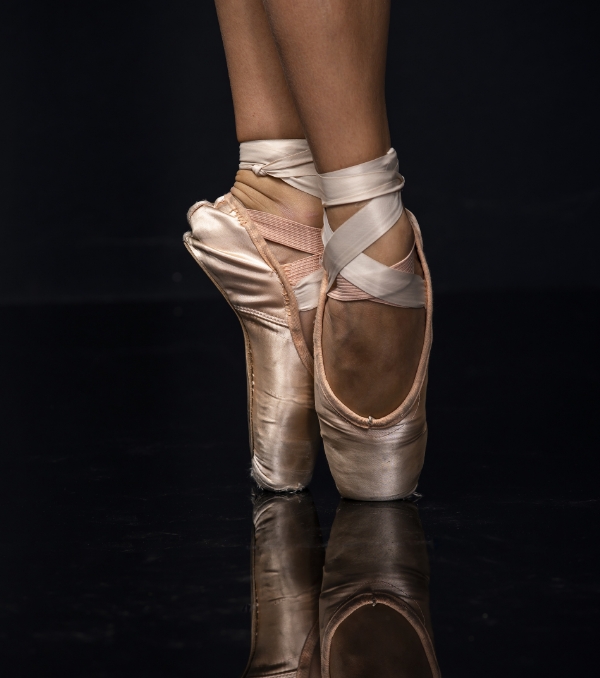This close-up photograph showcases a ballerina's feet positioned gracefully on pointe, adorned in worn pink satin ballet slippers. Her light brown or tan legs transition into tightly wrapped ankles, encircled by a mixture of cream-colored and pink satin ribbons, which criss-cross and tie the slippers securely in place. One foot is elegantly pointed forward while the other is slightly turned to the side, highlighting the dancer's flawless balance and poise. The highly polished black floor beneath mirrors the ballet slippers, amplifying the image's artistic appeal. The well-worn condition of the slippers is evident through the visible scuff marks, wrinkles, and creases, particularly at the toes and heels, suggesting they are well-used practice shoes. The black background enhances the dramatic focus on the ballerina's feet, capturing the intricate details of the satin ribbons, elastic bands, and the tension displayed in her tendons and extended pose.